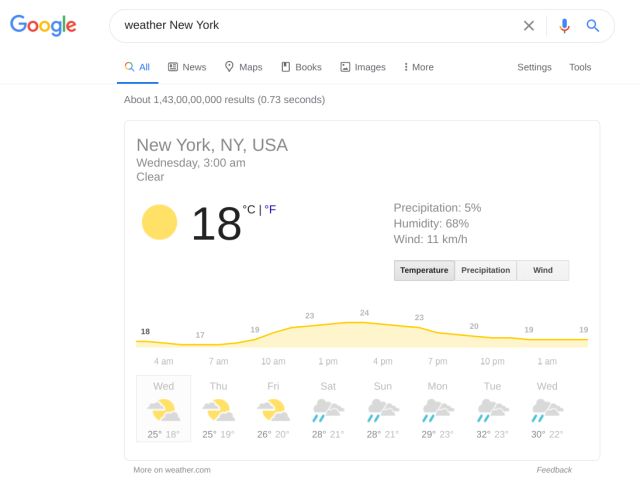A detailed screenshot of a Google search page, capturing a weather query for New York. At the top left, the recognizable Google logo is displayed, and the search bar at the top confirms the query with the text "weather New York." The majority of the screen is dominated by a detailed weather forecast graphic. 

At the top of the graphic, it indicates the location as "New York, New York, USA". The report details the day, which is Wednesday, and the time, 3:00 a.m., with a clear weather forecast currently. The current temperature is prominently displayed as 18°C, with an option to switch to Fahrenheit visible but not selected. To the right of the temperature, additional weather details are provided: a 5% chance of precipitation, 68% humidity, and wind speeds of 11 kilometers per hour.

Below these details, a chart presents the temperature forecast graphically over the course of the day, showing an early morning rise, peaking during late morning to afternoon, and dropping again in the evening. Further down, a multi-day forecast indicates that the next few days will start cloudy for the first two days, followed by potential rainfall two days after Wednesday.